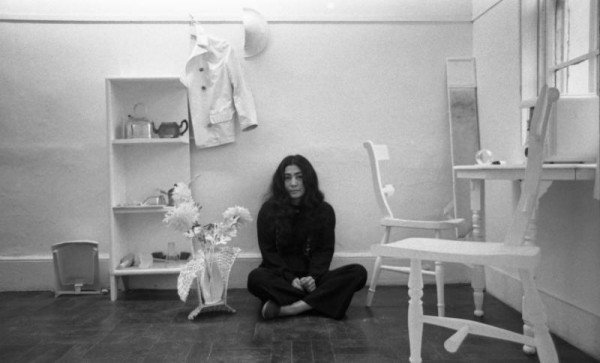This black-and-white photo features a woman dressed entirely in black sitting cross-legged on the ground with her hands clasped in her lap. She has long, straight black hair parted in the middle that cascades over her shoulders, and she gazes directly at the camera with a neutral expression. The setting appears to be a stark, minimalist room dominated by light elements. Behind her is a light-colored wall with a white coat, resembling a chef's coat, hanging on it. To the left of this coat is a narrow, white bookshelf-like structure with three shelves, each holding various small items. Positioned on the floor to her left is a vase containing white flowers. To her right are two white wooden chairs; one is facing a small white table, while the other faces away from it, creating a cozy but somewhat austere scene. The floor, contrasting the predominantly white room, is a slightly dusty gray hardwood, adding depth to the photograph while highlighting the woman who remains the central, striking figure in her dark attire.